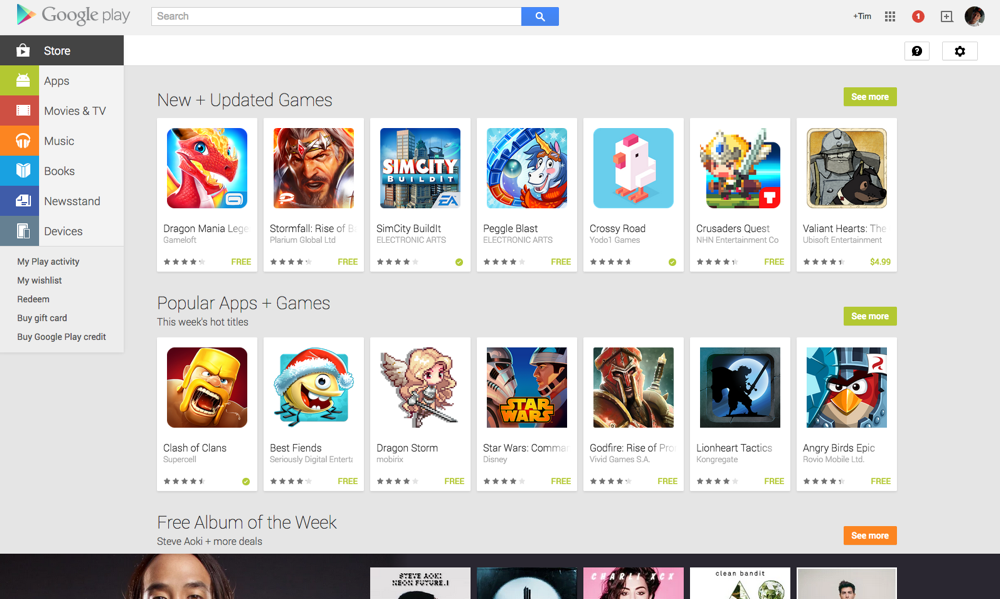In the upper left corner of the image, set against a grey background, is the familiar Google Play store button that features a multicolored triangle pointing to the right, rendered in hues of blue, yellow, and red. Adjacent to the icon, the words "Google Play" are displayed in grey. Below this, a white search box is visible.

On the right side of the search box, there is a small collection of icons: a "plus 10" indicator, a 3x3 grid of dots, and a red circle containing a white number "1." Next to these, a grey square with a plus sign in it is noticeable, and slightly obscured to the side is a small, round profile picture of the user.

Running vertically down the left side, black text on a white background lists categories: "Store," followed by "Apps," "TV," "Movies," "Music," "Books," "Newsstand," and "Devices." Underneath these categories, in smaller print, it reads: "My Play Activity," "My Wishlist," "Redeem," "Buy Gift Card," and "Google Play Credit."

On the right side of the image, a darker grey section is visible. At the top of this section, the text "New + Updated Games" is prominently displayed, followed by an orange button with white text that says "See More." Below this, several mobile game icons are displayed, described as overly simplistic and misleading in their representation. This section is followed by another heading, "Popular Apps & Games," also accompanied by a "See More" button, featuring more game icons that are similarly critiqued.

Towards the bottom, there is a mention of a "Free Album of the Week" featuring "Steve Akoli," accompanied by a "More Details" link and another "See More" button. The left side of this section has a black background, showing the top of someone's forehead, hinting at album covers positioned to the right.

The overall description captures the layout and elements of the Google Play Store interface, providing detailed insights into the various sections and visual components present in the image.